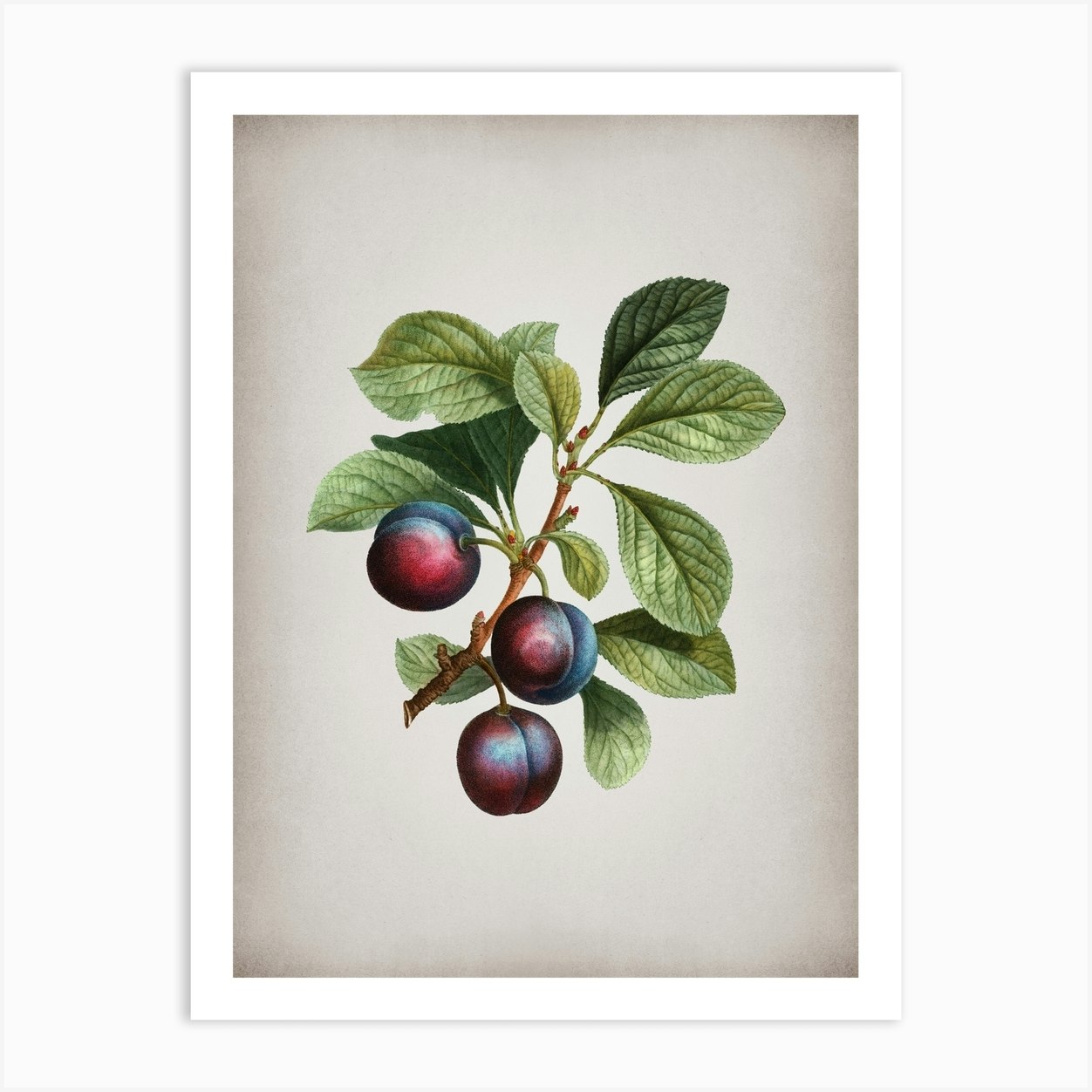This visually striking artwork, encased in a sleek white frame, features a detailed and realistic depiction of a plum tree branch rendered in colored pencils or possibly paint. Against a very light beige or grayish off-white backdrop, the central focus is a medium brown branch, which appears as if it has been freshly snipped from a tree. Hanging from this picturesque branch are three plump, somewhat shiny plums characterized by their deep purple hues with subtle hints of pink. The plums exhibit a natural sheen with light reflecting off their closest facets. Surrounding the plums are an array of green leaves, possibly numbering around ten or twelve, sprouting from various points along the branch. At the top end of the branch, a tight cluster of leaves emerges from small buds, adding to the richness and authenticity of the depiction. The botanical elements are vividly portrayed, giving the artwork a lifelike presence, with careful attention to the light interacting with the textures and colors of the plums and leaves. The entire composition is centered meticulously within the frame, drawing the viewer's eye to the harmonious balance of nature captured within the artwork.